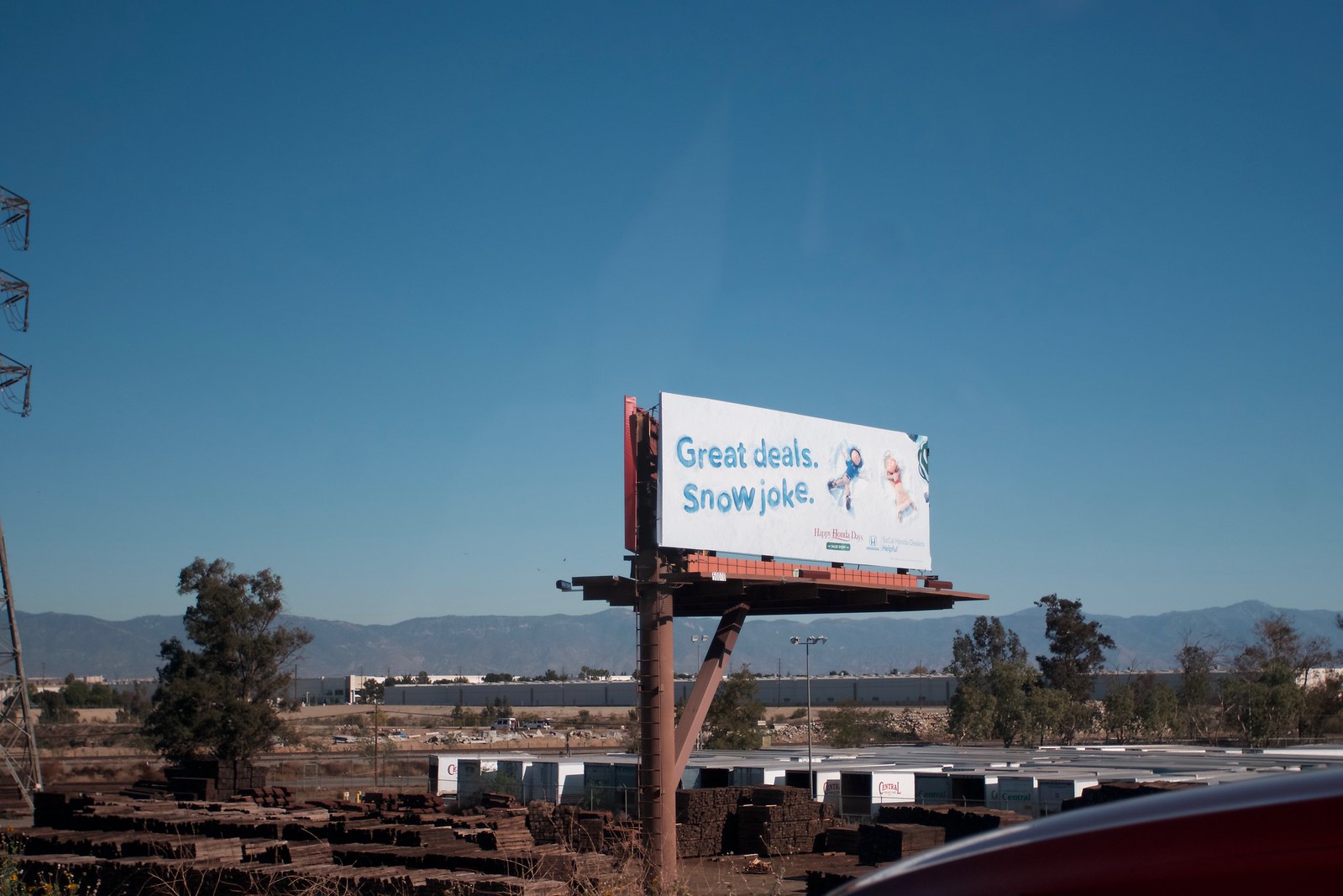The image showcases an elevated, older billboard perched atop a thick brown post with a boxy support extending from it. The billboard features a white background with the text "Great Deal Snow Choke" prominently displayed. Beneath the text, there is an indistinct image of two individuals, one wearing a blue shirt and the other in a red shirt, though the details are too distant to discern clearly. The backdrop is a brilliantly blue sky with rugged mountains visible in the distance, sectioned off by the horizon. The photo appears to have been taken from inside a vehicle, as indicated by a part of the car visible in the lower right-hand corner. The scene also includes a skyline of truck trailers parked in storage, with several piles of hay and a cluster of warehouses visible in the background. A cell tower is situated on the left side of the image, adding to the industrial ambiance of the setting.